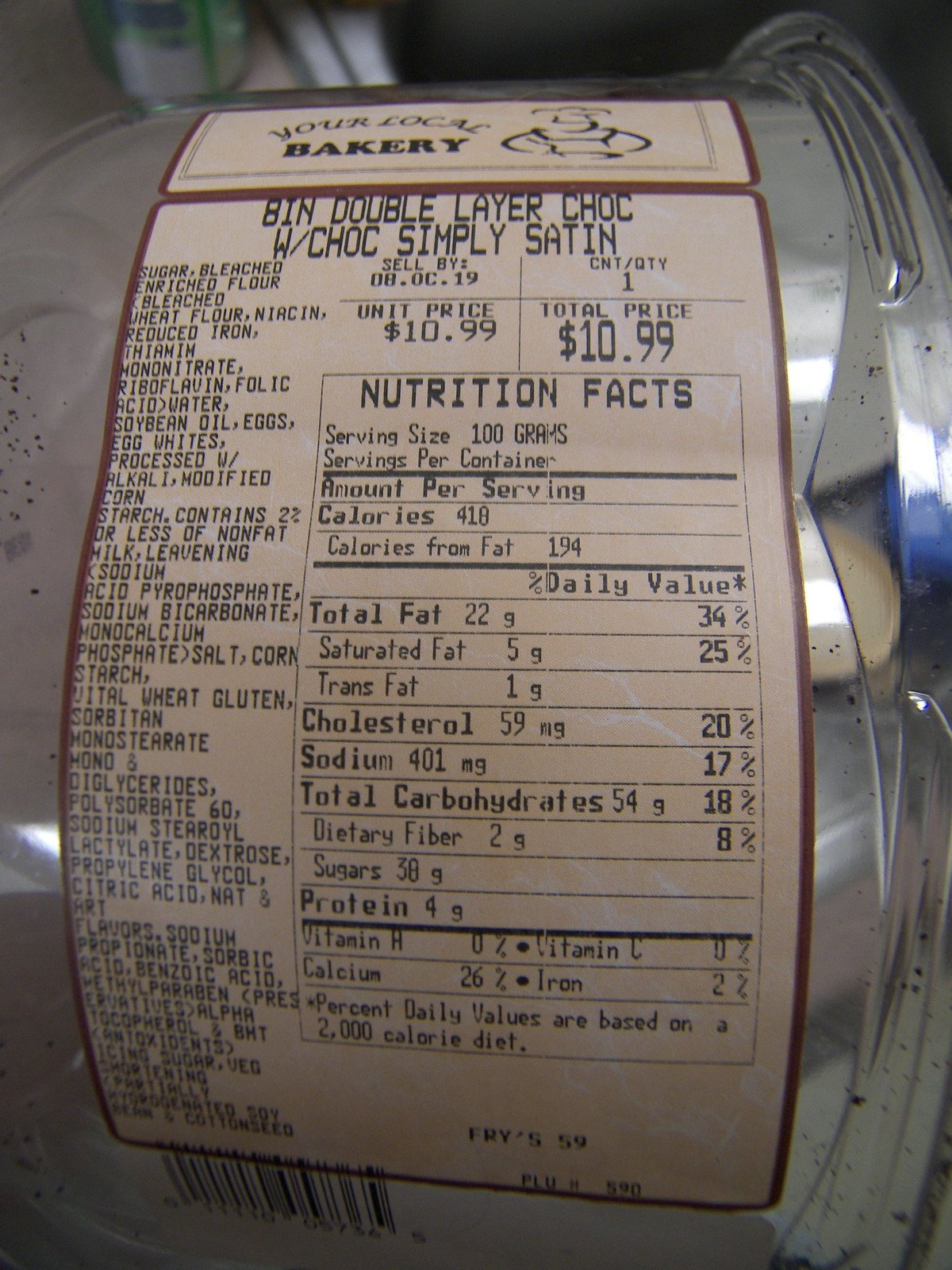Here is the cleaned-up and detailed caption for the image:

---

This image showcases a delectable double-layer chocolate cake from a local bakery. The cake is adorned with a smooth chocolate satin icing. A beige label, outlined in brown, is visible on the packaging. It reads, "Your Local Bakery" at the top and provides key details, including the price of $10.99. The label also includes detailed nutrition facts: each 100-gram serving has 410 calories, with 194 calories derived from fat. The total fat content is 22 grams, making up 34% of the daily recommended value, while the saturated fat content is 5 grams, accounting for 25% of the daily value.